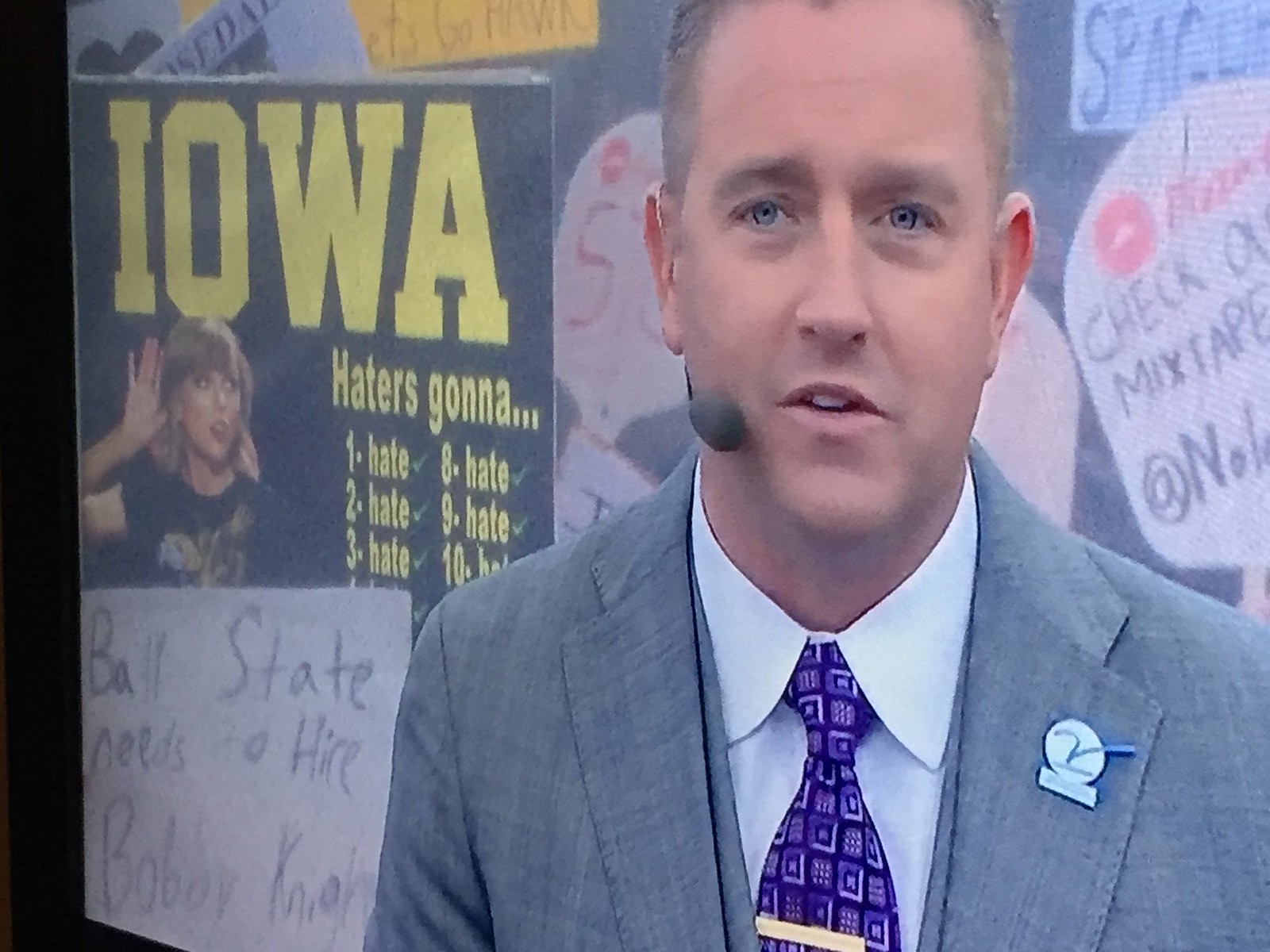In the image, a sports announcer stands prominently in the center, facing the camera, wearing a light blue suit, a dark blue tie, and a white shirt. He has a wraparound earphone microphone positioned near his mouth and a pin with an insignia on his left lapel. The background is filled with various handwritten signs in different colors.

To the left of the announcer, a large black banner features bold yellow letters spelling "Iowa" at the top-left. Directly below the "I-O" of "Iowa" is a picture of Taylor Swift with her hand raised to her ear as if listening. Adjacent to her image, the banner quotes lyrics in yellow text: "Haters gonna hate, hate, hate, hate, hate, hate." Below this, there is a handwritten white poster board stating, "Ball State needs to hire Bobby Knight."

In addition, there are other visible signs: to the right of the announcer, someone holds up a white sign reading "Check our mixtape," and behind that, another sign partially visible with "Spaghetti" or "S-P-A-G" written on it. Above the black "Iowa" poster, a yellow sign says "Go Hawks." Behind and around these, more handwritten signs in blue, yellow, and white can be seen, contributing to a lively and colorful backdrop.